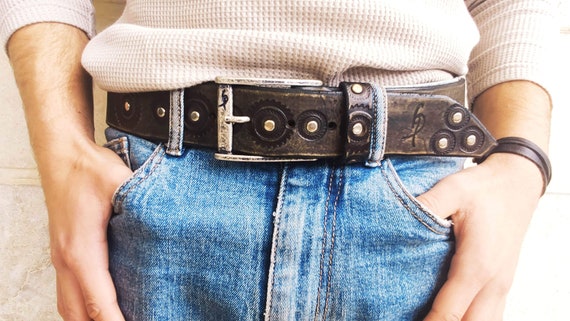The photograph captures the midsection of a model, focusing on the attire and specific accessories. The model, who could be either male or female, is wearing blue jeans with a rustic-looking, wide black leather belt adorned with silver studs that encircle the belt. The belt features a notable silver buckle that secures it through the visible holes. Above the belt, the model has tucked in an off-white, long-sleeved shirt with a subtle, small square pattern; the sleeves are slightly pulled up, exposing some black hair on the lower arms. Both thumbs are casually hooked into the front pockets of the jeans, adding a relaxed vibe to the pose. On the right wrist, the model sports a brown leather bracelet, which complements the overall rugged aesthetic of the ensemble. Only a small portion of the area just above the belt is visible, emphasizing the detailed texture and style of the clothing and accessories.